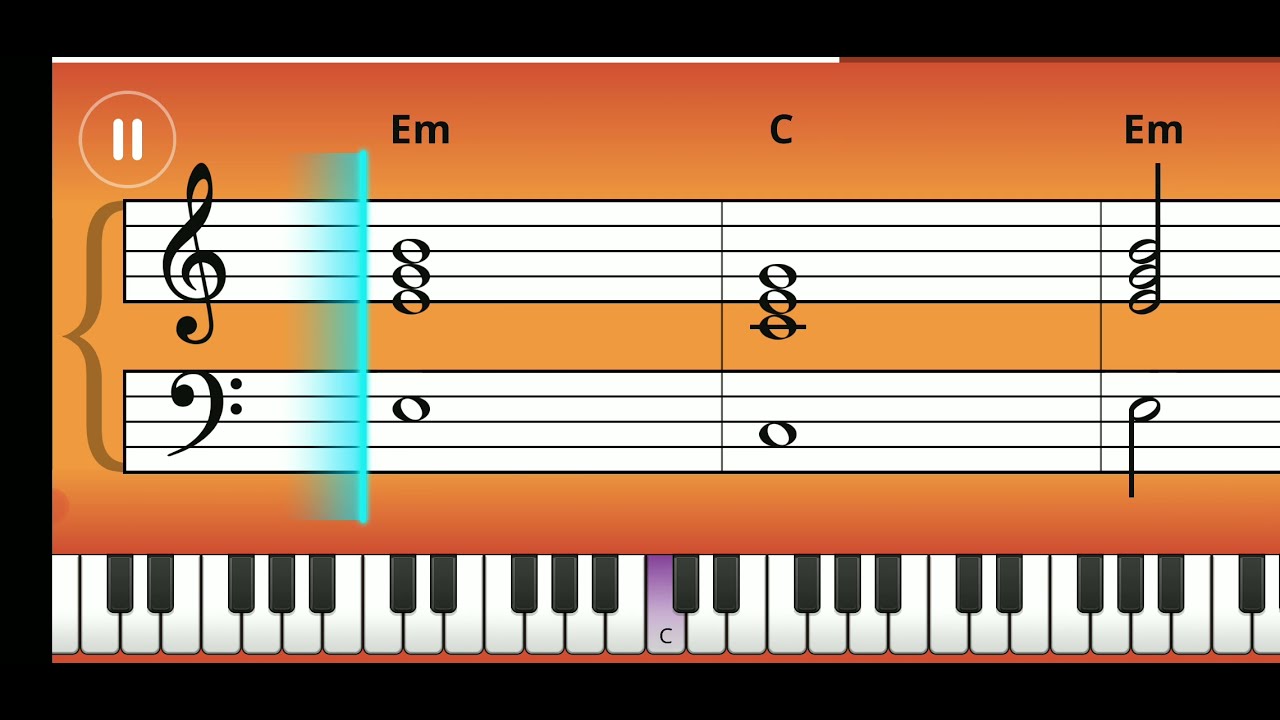The image is a screenshot of a digital piano keyboard app set against an orange gradient background. At the top left corner, there's a pause button inside a circle. Below the pause button, there's a blue progress bar indicating the playback position on a music sheet. The sheet music displays both treble and bass clefs with the notation for E minor (E-M), C, and E minor (E-M), followed by corresponding whole, half, and quarter notes. The keyboard itself is depicted at the bottom, with all the keys shown, and the middle C key highlighted in purple. The app appears to be a piano lesson video, guiding users through the notes and keys to play.